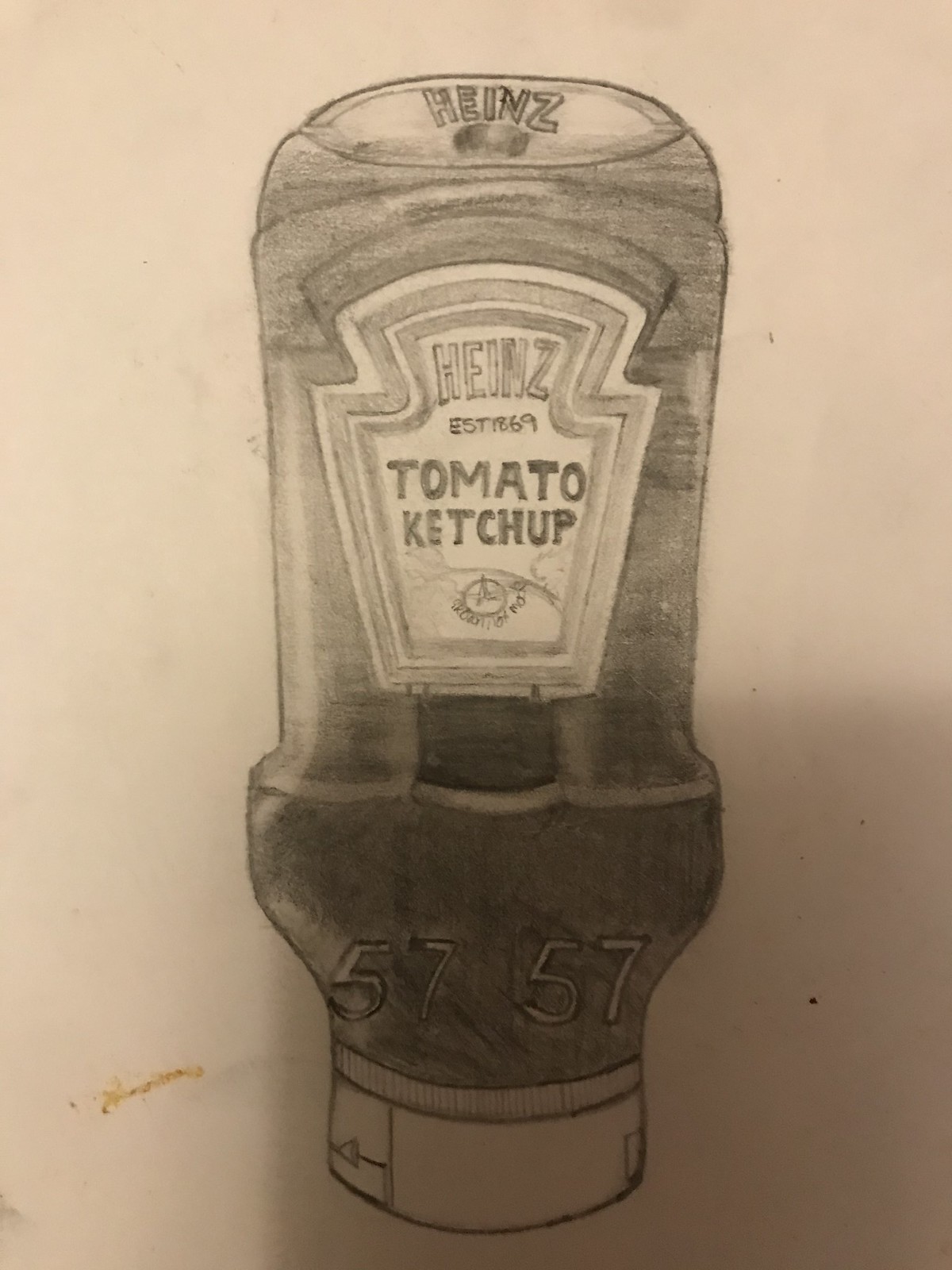This detailed pencil drawing portrays an inverted plastic bottle of Heinz Tomato Ketchup, meticulously rendered on off-white paper. The shadow cast on the lower right quadrant of the paper adds depth and realism to the artwork. The bottle is depicted upside down, with the cap at the bottom, ensuring the label is oriented correctly. The label prominently showcases the iconic Heinz logo, including "Heinz Established 1869" and "Tomato Ketchup." At the top of the drawing, which represents the bottom of the actual bottle, the word "Heinz" is embossed within a plastic oval base. The white plastic cap, featuring a ribbed rim, is precisely illustrated with the number "57" appearing twice at the bottom, capturing the essence of this everyday household item with remarkable attention to detail.